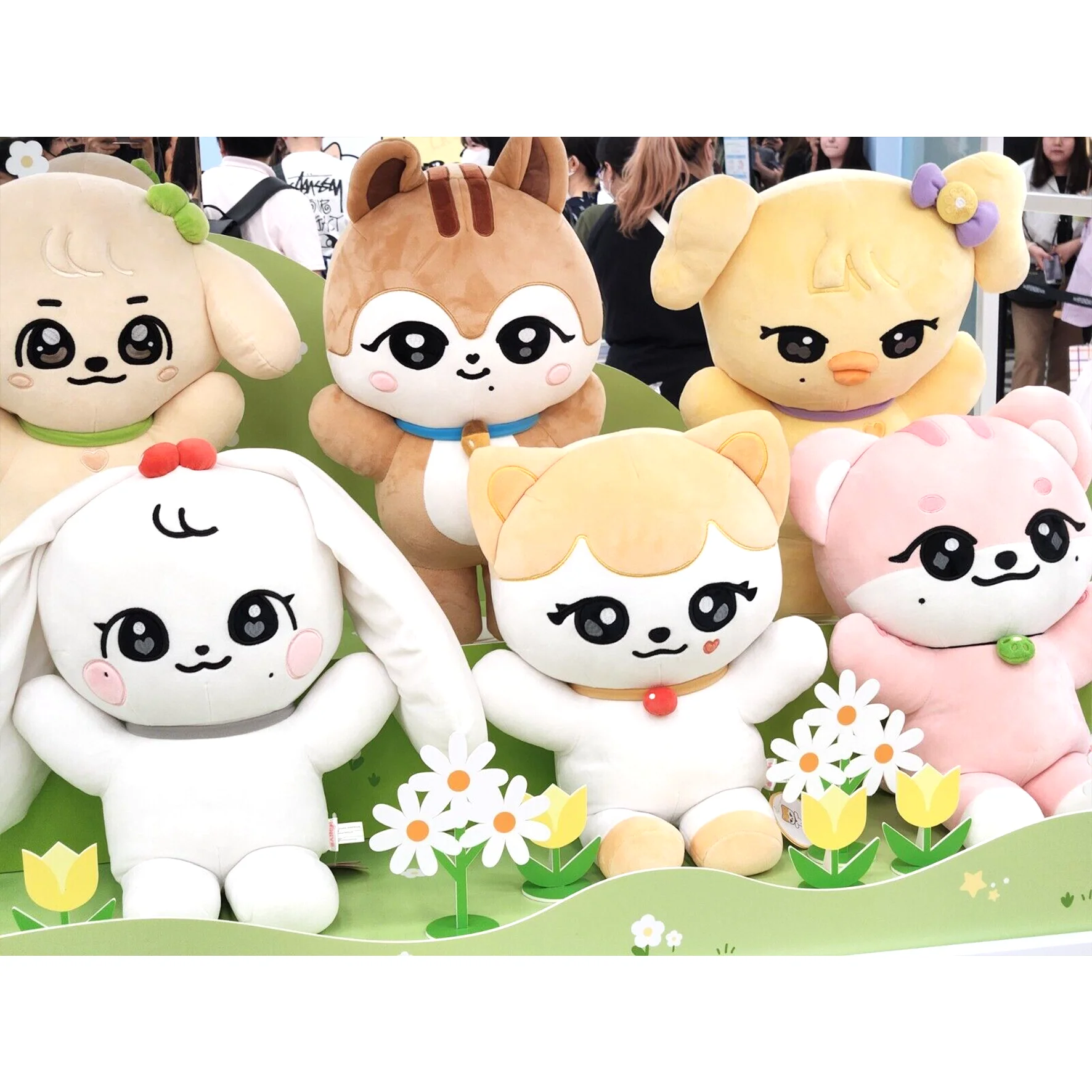A delightful scene showcases six adorable plush animals nestled in a green box adorned with painted flowers, including yellow tulips and white daisies. Starting from the lower left, the first plush is a white bunny rabbit with long ears, pink cheeks, hearts in her eyes, and little red balls atop her head. Next to her is a charming white kitty cat featuring yellow hair, yellow ears, a heart-shaped beauty mark, and a red ball on an orange collar. Amidst the plushies are more flowers, leading to a pink teddy bear with white accents on its ears, mouth, and feet, sporting a green ball necklace. 

At the upper left, a cream-colored dog with rosy cheeks wears a green collar and a matching green bow on its head. Beside the dog is a chipmunk (or squirrel) plush with brown stripes on its head, white facial markings, a light brown body, and a blue collar. Finally, on the right side, a yellow chick-like creature with an orange beak, ears, and a purple bow adds to the cuteness. These plush animals, each with unique characteristics and big, expressive eyes, create a charming and heartwarming tableau.